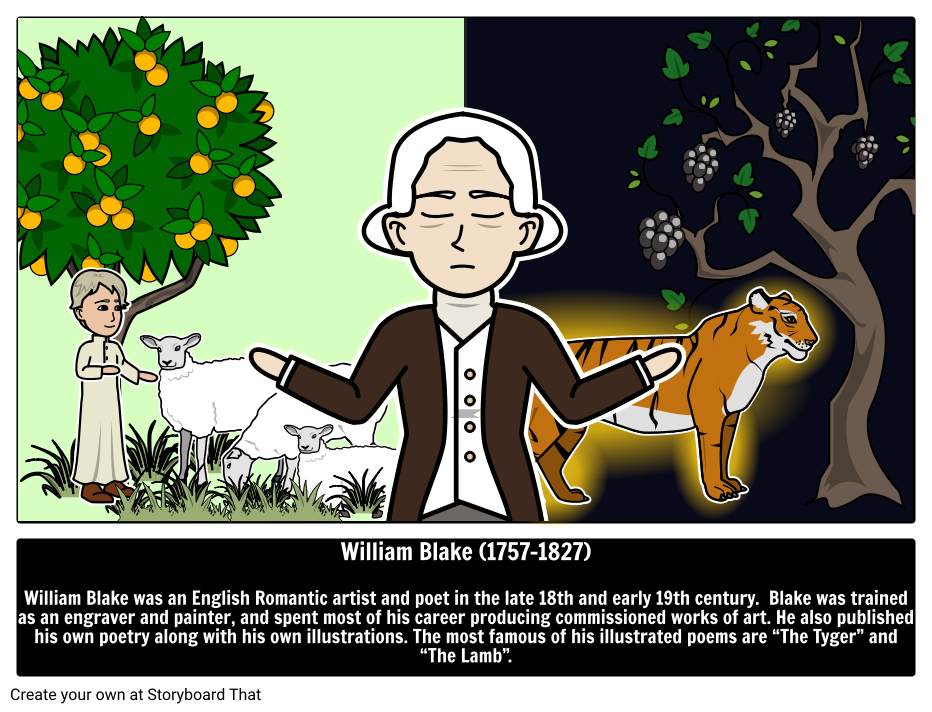The image is a hand-drawn storyboard slide that depicts two scenes under the name William Blake (1757-1827), an English Romantic artist and poet known for his illustrated poems "The Tiger" and "The Lamb." On the left-hand side of the image, set against an olive light green background, there is an elderly man with gray hair, dressed in a beige robe with two buttons, and light brown boots, reaching towards a sheep. This sheep, like the other two beside it, has a gray face, a white coat, and gray legs. The man stands beneath a dark brown tree with a mix of dark green and light green leaves, as well as oranges highlighted with light brown accents, while light green grass shoots up sporadically. Behind this scene, another image shows the same elderly man wearing a white undershirt with yellow buttons and a brown vest, extending his arms. 

On the right-hand side, a contrast is set with a black background featuring an orange Bengal tiger with black stripes, a white underbelly, ears, and fur below its chin. The tiger stands beside a tree that has a light brown trunk, dark and light green leaves, and what appear to be gray and black berries. 

At the bottom of the image, white text on a black rectangle reads: "William Blake, 1757 to 1827." Below it is a brief biography stating, "William Blake was an English Romantic artist and poet in the late 18th and early 19th century. Blake was trained as an engraver and painter and spent most of his career producing commissioned works of art. He also published his own poetry along with his own illustrations. The most famous of his illustrated poems are The Tiger and The Lamb." Additionally, there is a prompt to “create your own storyboard” at storyboardthat.com.